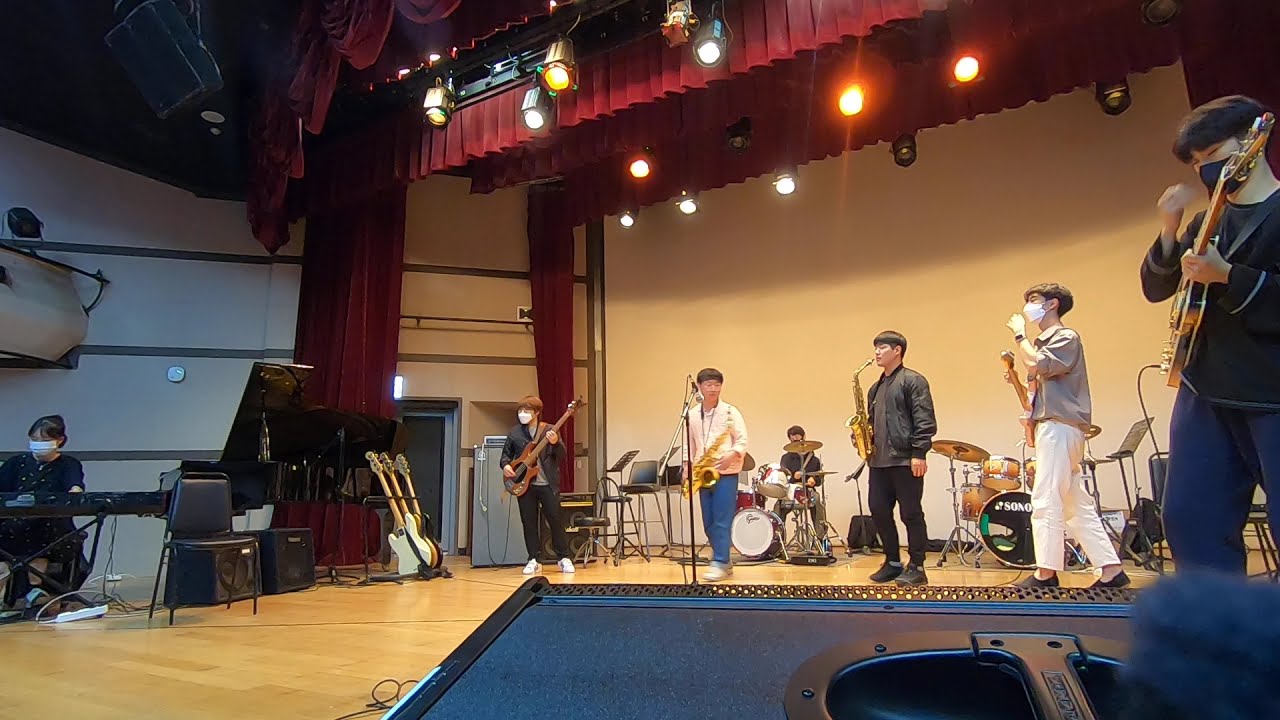This image captures a band, seemingly composed of youthful music students, performing on a classical stage adorned with maroon red curtains and sophisticated lighting rigs. Seven individuals are arranged predominantly to the right of the stage, with one female guitar player slightly separated to the left. The members, who appear to be Japanese based on their features, wear a variety of colored pants—white, black, and blue—and shirts in shades of white, black, and gray, contributing to a cohesive yet casual appearance.

In the front row, closest to the camera, is a guitar player dressed in a black sweatshirt with white stripes, playing a brown and black guitar. To his left, another person in white pants and a tan long-sleeve shirt holds a guitar, though not actively playing it. Immediately next to him stands a saxophone player with a microphone, followed by another saxophonist without a mic. Moving further to the right is a bass player, adding depth to the rhythmic section. Behind the saxophone players, slightly to the right, sits an open drum set, bearing the brand name Sono—its drum shells colored in striking gold and black tones, alongside another set in red and white hues.

To the far left, a woman operates a keyboard, contributing to the harmonic baseline of the ensemble. The stage itself features a light wood floor, and a black speaker is positioned at the very bottom of the image, just visible from the camera's perspective. This scene is clearly set in an auditorium, illustrating an engaging practice session or impending musical performance.